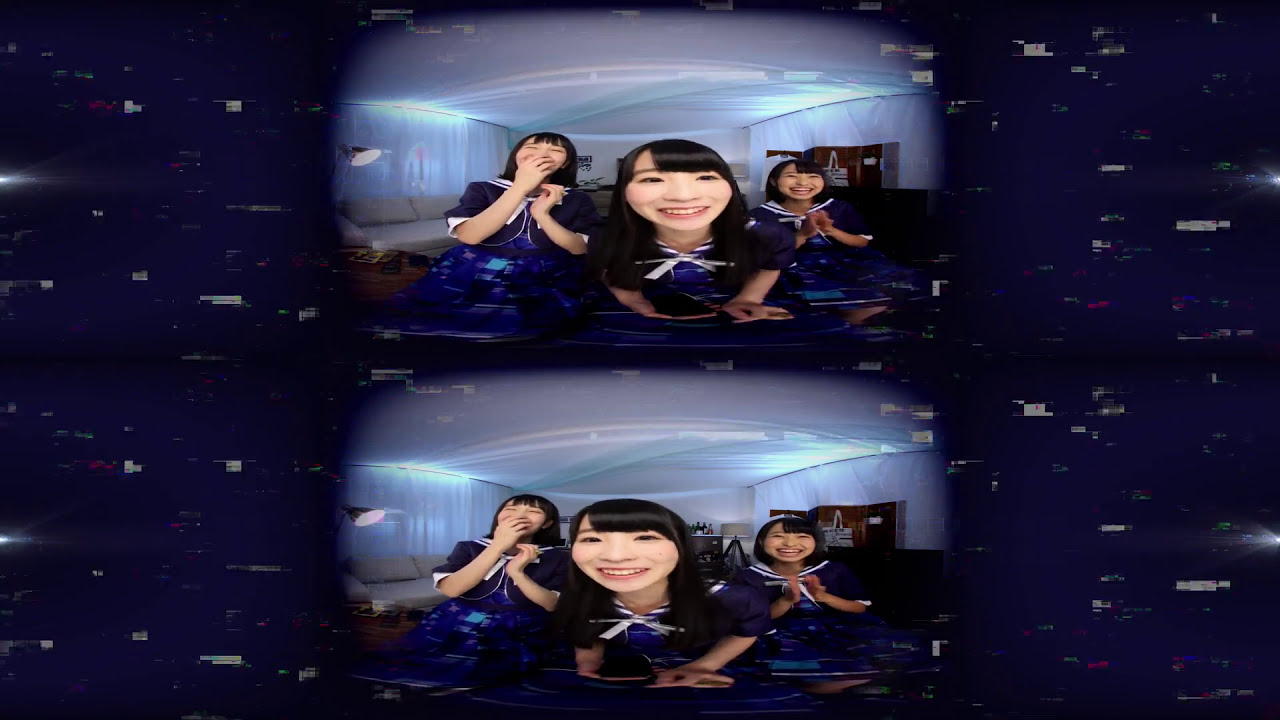This image is a collage consisting of two sets of the same photograph arranged one above the other, featuring three young girls. In both sets, the girl on the left is of East Asian descent, with shoulder-length hair that covers her ears and bangs that stop just above her eyebrows. She's wearing a dark blue shirt with white lines and is captured mid-laugh, covering her mouth with one hand and has the other close to her chin. The girl in the center has brown eyes and straight hair similarly cut with bangs just below her eyebrows, parted slightly to reveal her forehead. She's smiling broadly, showing her upper teeth, and also wears a dark blue shirt with a blue line down the center. Notably, in the top photo, she is looking to the right, while in the bottom one, she’s looking to the left. The girl on the right mirrors the cheerful atmosphere, smiling brightly with her teeth visible and her hands up, seemingly clapping. She also has bangs and wears the same style blue shirt as the other two girls. All of them seem to be enjoying themselves, radiating a sense of joy and camaraderie. The background includes a ceiling with streaks of green and yellow lights, and additional details like curtains, lamps, and a TV can be seen, suggesting the photo was taken indoors. The overall color palette of the collage includes blue, black, white, green, and minor accents of tan and silver, lending a vibrant yet intimate feel to the setting.